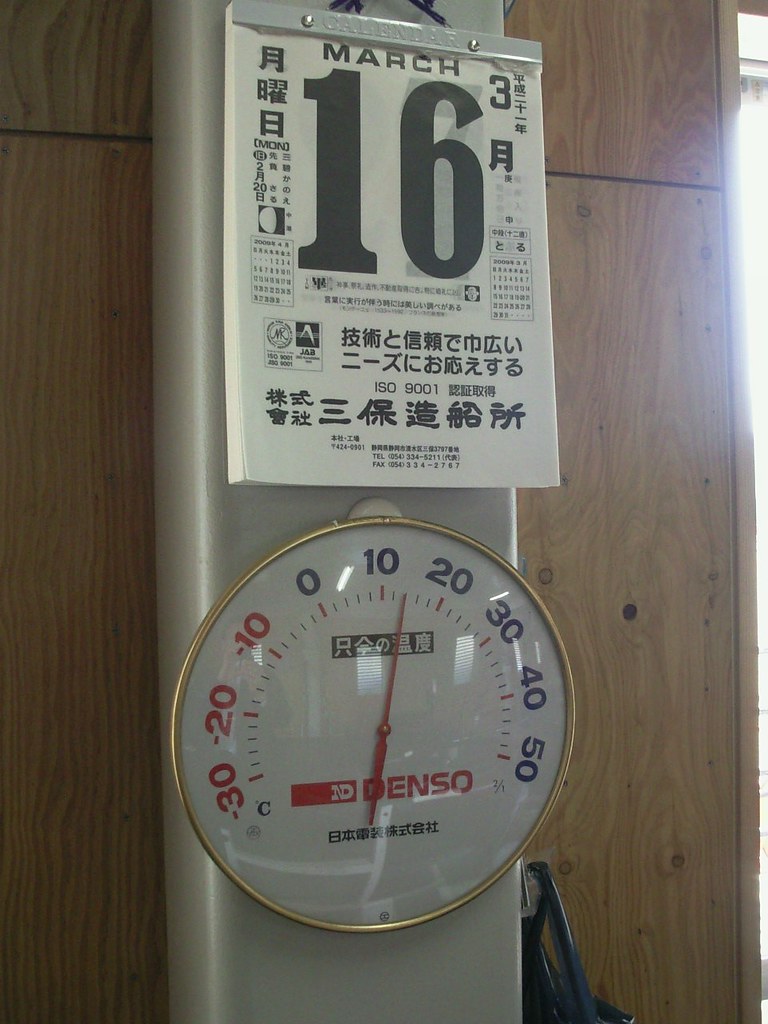The photograph, captured in portrait orientation, provides an insightful glimpse into a Japanese setting, potentially a shop or another indoor space in Japan. Dominating the image is a tall, rectangular metal structure, placed against a panelled wall featuring a wood grain texture. Mounted on this vertical pole, a printed calendar is prominently displayed at the top.

The calendar, hanging from a black string that extends just out of frame, indicates the date as March 16th. The month "March" is printed in smaller text at the top, while the number "16" is displayed in large, bold black numerals. The calendar is adorned with traditional Japanese characters and features a side profile that reveals the stacked pages of upcoming days.

Beneath the calendar, an analogue thermometer hangs, marked with a red needle that currently points two increments past the 10, positioned where 12 o'clock would be on a clock face. The thermometer also displays Japanese characters and carries the brand name "Denso" (D-E-N-S-O) in English. Encircling the thermometer's glass or plastic front, there is a golden bezel reflecting light and details of the surrounding environment. Notably, the bezel includes a clear reflection of the photographer. The reflected image shows two hands holding a smartphone in portrait orientation, aligning with the format of the photograph.